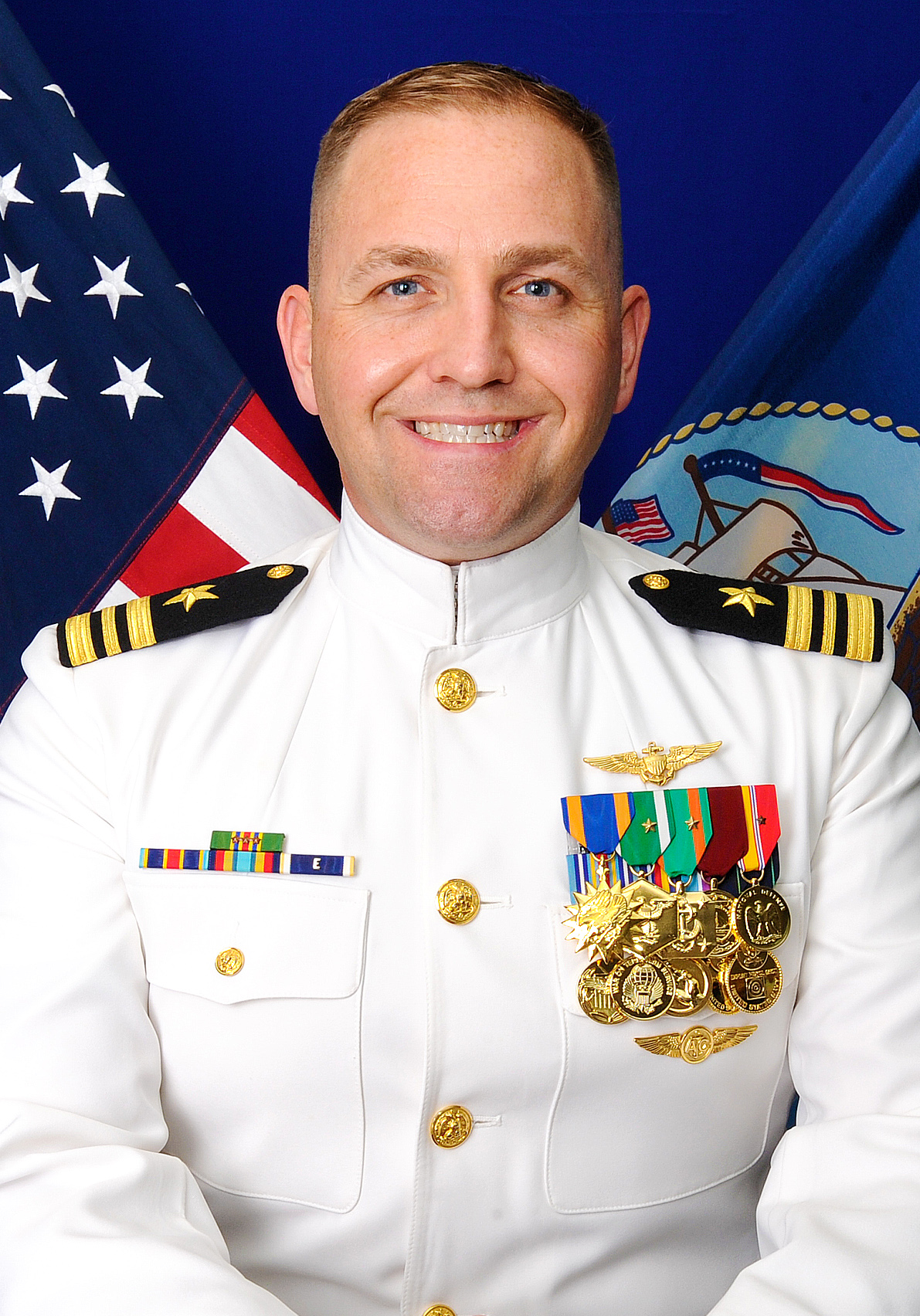This photograph depicts a proud Caucasian man, likely in his mid-30s to 40s, grinning broadly with immaculate white teeth. This individual, presumed to be a Navy officer due to his regalia, has striking light blue eyes and very short-cropped blonde hair. He is dressed in a pristine white military uniform adorned with gold buttons. On his shoulders, there are dark navy blue epaulets that feature gold stars and three yellow stripes. 

His left breast pocket showcases a plethora of medals and badges of various sizes and shapes, predominantly gold and meticulously polished to a high sheen. The collection includes at least nine distinct medals, some circular and one notably resembling a sun, indicating a rich history of achievements.

The background features a patriotic display with multiple flags. To his right, there is a glimpse of an American flag with its stars and stripes, while to his left, parts of another flag are visible, which appears to have a design reminiscent of a boat and eagle, and a stretched-out American motif. The backdrop behind his head is a deep blue. This image exudes his pride and dedication to his service.